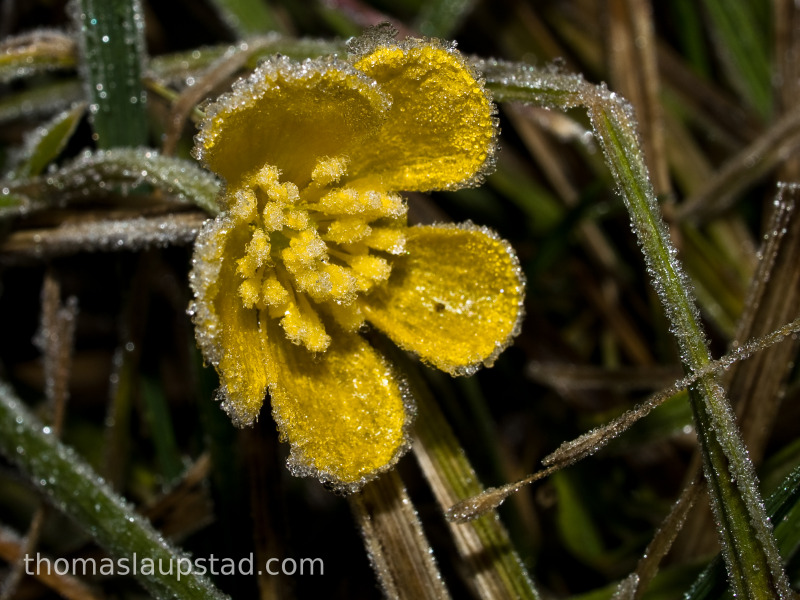This image is a close-up shot of a tranquil and beautiful yellow flower, slightly off-center to the left against a background of green and brown blades of grass and branches. The photo has a calming, almost ethereal quality, with silver dew-like droplets delicately adorning the foliage and flower, giving the appearance of a soft, silvery fuzz. The flower itself, with its vibrant yellow petals, radiates from a brown stem, and contains a cluster of around 15 smaller yellow buds at its heart. Each element, including the surrounding grass and branches, is covered in what looks like a sprinkle of tiny silver droplets, adding to the serene atmosphere of the image. The bottom left-hand corner features the text "Thomaslobstad.com" subtly integrated into the composition.